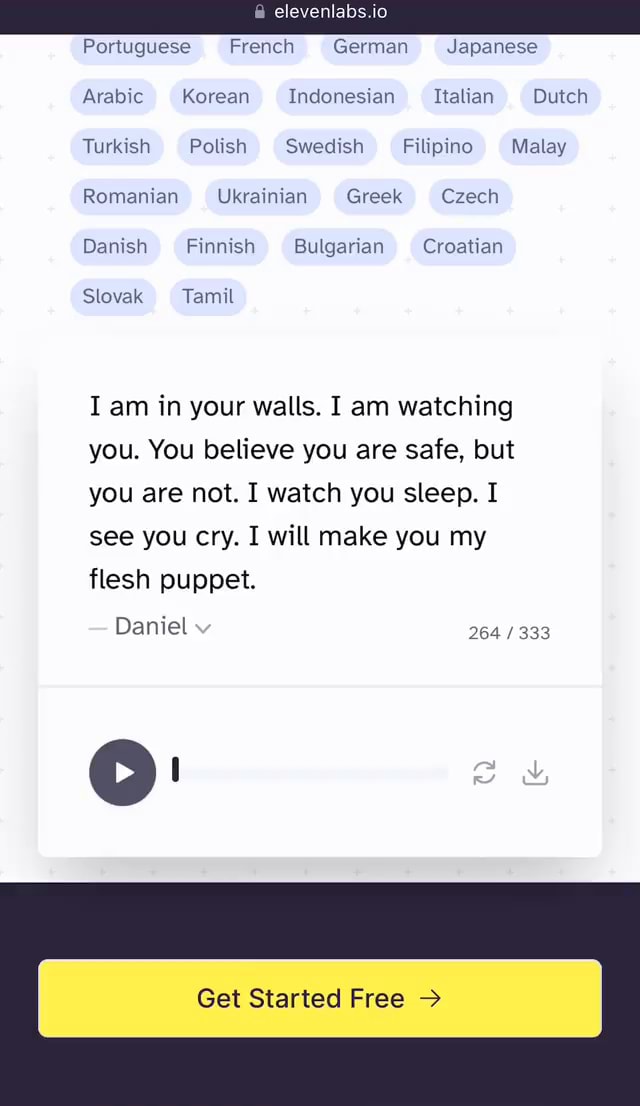This image is a screenshot from the website 11labs.io. At the top, the website's name is displayed in black text with a white font, accompanied by a light gray padlock icon to the left, indicating a secure site. The website's background is predominantly white, featuring several light blue buttons with black text, each representing different languages. The buttons are organized in multiple rows and include languages such as Portuguese, French, German, Japanese, Arabic, Korean, Indonesian, Italian, Dutch, Turkish, Polish, Swedish, Filipino, Malay, Romanian, Ukrainian, Greek, Czech, Danish, Finnish, Bulgarian, Croatian, Slovak, and Tamil.

In the center of the image, there is a white text box with a chilling message written in black font: "I am in your walls, I am watching you, you believe you are safe, but you are not, I watch you sleep, I see you cry, I will make you my flesh puppet." This text is attributed to "Daniel," written in light gray, followed by a downward-pointing arrow. The character count is shown in the bottom right corner of the text box, displaying "264 out of 333" in light gray.

Below the text box, there are several dark gray icons: a right-pointing arrow resembling a play button, a replay button, and a download button, indicating interactive features. Further down, a purple block with a prominent yellow button is visible, marked with the text "Get started free" and an arrow pointing right, suggesting a call to action for new users. This screenshot seems to be from a translation app available on the website.